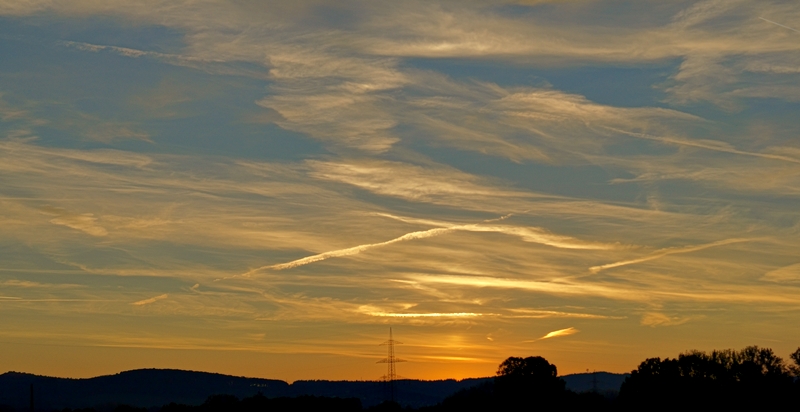This image captures a breathtaking sunset or sunrise scene, with the sky dominating most of the frame. The backdrop reveals a dark blue sky with wispy white and streaked clouds that blend into hues of yellow and orange as they approach the horizon. The sun, positioned near the center-bottom, is either setting or rising against a silhouette of a forested area, with trees primarily located on the bottom right of the image. To the left of the trees, a cell tower partially obscured by the forest peaks into view. The colors present in the scene range from blues and whites in the sky to greens and browns for the trees, creating a harmonious natural setting. There are no buildings or text in the image, suggesting it was taken in a rural location, likely during the summer given the warm tones and inviting atmosphere. Overall, the photograph exudes a serene beauty, capturing a moment of natural splendor.